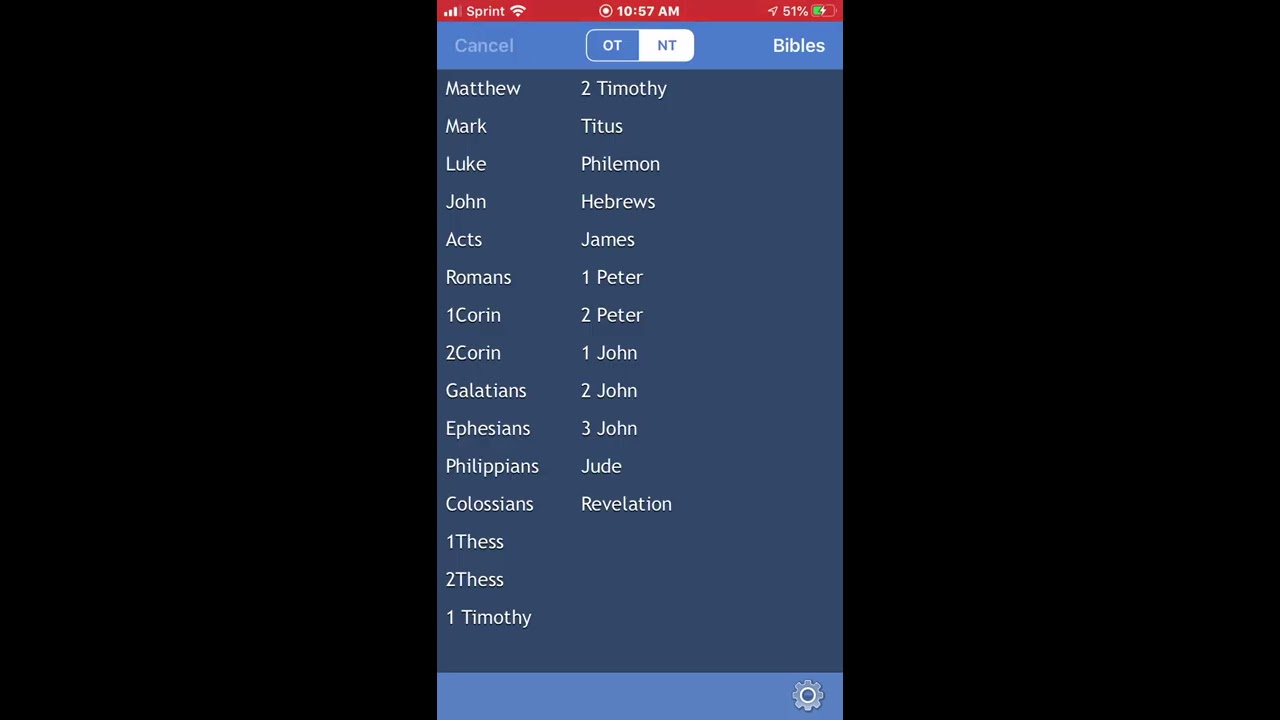The image depicts a screenshot of a cell phone screen with a dark blue background. At the top of the screen, there's a red status bar indicating the carrier "Sprint," signal strength bars, Wi-Fi connection, the time "10:57 AM," and a battery level of "51%". Just below this is a blue banner featuring a "Cancel" button on the left, the abbreviation "O.T." and "N.T." centered, with "N.T." selected and highlighted in white, and the word "Bibles" on the right. The main portion of the screen displays a list of New Testament Bible books in white text on a navy background, organized into two columns. The left column lists: Matthew, Mark, Luke, John, Acts, Romans, 1st Corinthians, 2nd Corinthians, Galatians, Ephesians, Philippians, Colossians, 1st Thessalonians, 2nd Thessalonians, and 1st Timothy. The right column lists: 2nd Timothy, Titus, Philemon, Hebrews, James, 1st Peter, 2nd Peter, 1st John, 2nd John, 3rd John, Jude, and Revelation. Black panels flank both sides of this central menu.